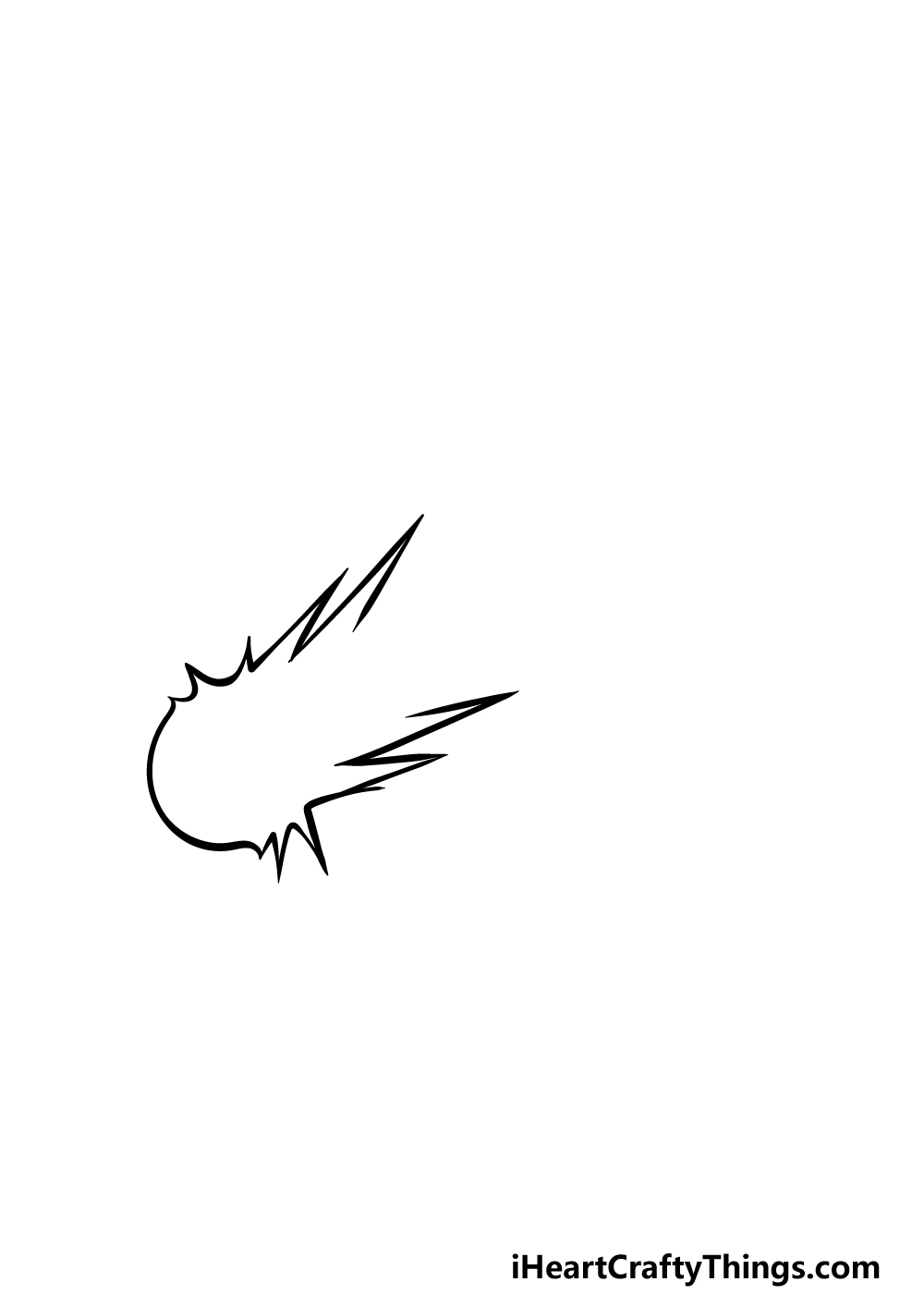The image is an abstract black and white illustration featuring a dynamic, jagged design. The main shape starts at the top with a rounded, half-circle arch and then extends into sharp, pointed lines that stretch downwards, creating an impression of a comet or lightning bolts, adding a sense of action and motion. The two main lines, jagged and irregular, are positioned at the left and right sides and taper off towards the bottom, leaving a significant amount of blank white space between them. The entire design is set against a white, open background without any enclosing borders, especially open on the right edge. At the very bottom of the image, there is a website URL written in lowercase black letters except for the capital letters "I," "C," and "T" in the words "I heart crafty things dot com," which indicates the possible source or creator of the artwork.